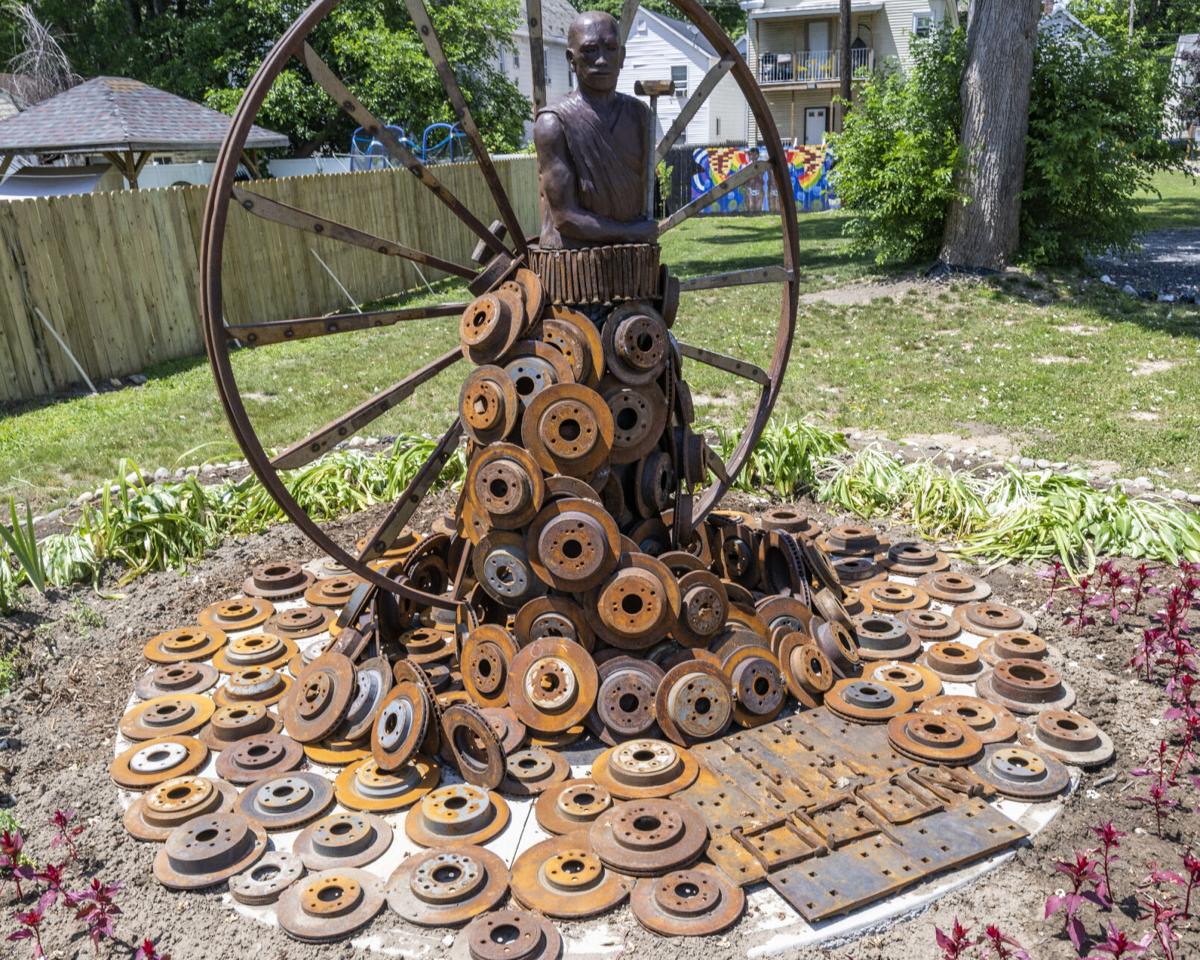In this full-color, square photograph, taken outdoors on a sunny day using natural light, we find ourselves in a sizable backyard within a neighborhood, framed by a wooden fence that separates the yards. Occupying the upper right corner, a large tree trunk and surrounding bushes add to the lush feel of the scene. Stretching across the top from the center to the upper left corner, white houses peek into view. There’s even a glimpse of a gazebo in a neighbor’s yard to the left.

The main attraction of the photograph is a striking sculpture, believed to represent John Henry. This impressive bronze figure is of a muscular Black man wielding a sledgehammer, his stance powerful and dynamic. Behind him stands a large metal wagon wheel, its goldish-brown hue weathered by rust. Scattered around the sculpture are numerous steel circular forms, resembling oversized washers, some laying flat on the ground and others stacked and ascending up the side of the statue.

The foreground features a circular dirt area bordered by low-cut palm leaves and dotted with small red or purple plants, adding vibrant touches to the earth-toned setting. The middle ground showcases patches of green grass interspersed with rocks and dirt, completing the natural yet artfully arranged environment. This photograph captures not just a backyard, but a thoughtfully curated outdoor space showcasing a unique and captivating steel sculpture under the bright midday sun.